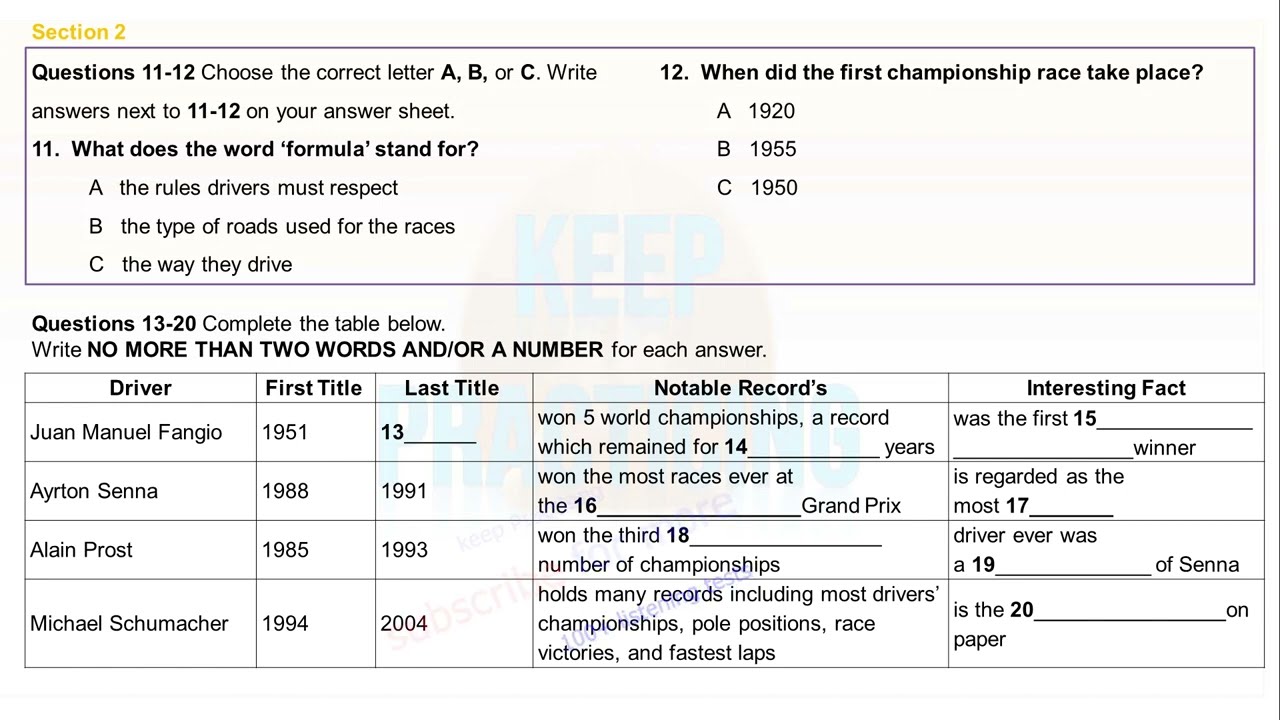The image depicts a written test page, primarily white with some yellow and gray accents. The top of the page is labeled in yellow text as "Section 2." Directly beneath is a gray box containing instructions and questions. The instructions state: "Questions 11 to 12. Choose the correct letter, A, B, or C. Write answers next to 11 and 12 on your answer sheet." The multiple-choice questions within this section are as follows: 

11. "What does the word formula mean?" with options:
   A. The rules drivers must respect
   B. The type of roads used for races
   C. The way they drive
   
12. "When did the first championship race take place?" with options:
   A. 1920
   B. 1955
   C. 1950

Below this, another instructional prompt states: "Questions 13 to 20. Complete the table below. Write no more than two words and/or a number for each answer." The table is divided into five columns labeled: "Driver," "First Title," "Last Title," "Notable Records," and "Interesting Facts," with multiple rows ready to be filled out by the test taker. Notable drivers like Juan Manuel Fangio, Ayrton Senna, Alain Prost, and Michael Schumacher are listed. In the background, there is a faint red watermark with partially visible text, appearing to say "keep."